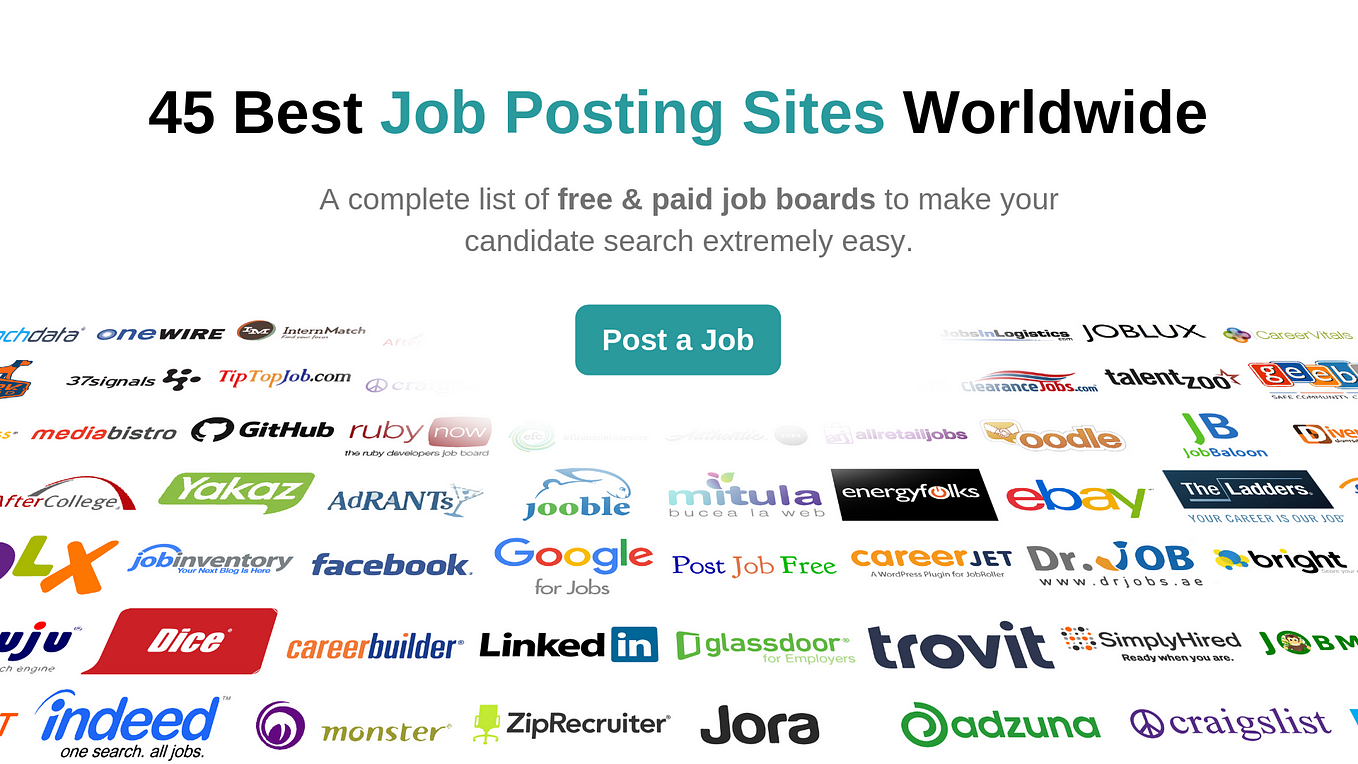A detailed screenshot of a job board aggregate website is displayed on the screen. At the top of the page, a prominent header reads "45 Best Job Postings Worldwide: A Complete List of Free and Paid Job Boards." This indicates that the site compiles various job boards to facilitate an efficient job search process for employers. Just below the header, there is a call-to-action button labeled "Post Your Job," which appears slightly more than a third of the way down the page. This section is designed for employers to click and submit their job listings.

Further down the page, the website features a comprehensive list of job posting sites, showcasing platforms where employers can advertise vacancies. The list includes popular and specialized job boards such as GitHub, Ruby, Jubal, Energy Folks, Dr. Job, ZipRecruiter, Monster, and Indeed. Each job board is likely accompanied by links or summaries, providing easy access for employers to explore and utilize these resources through the aggregate site. The overall design and layout are aimed at making the candidate search process extraordinarily convenient for employers.